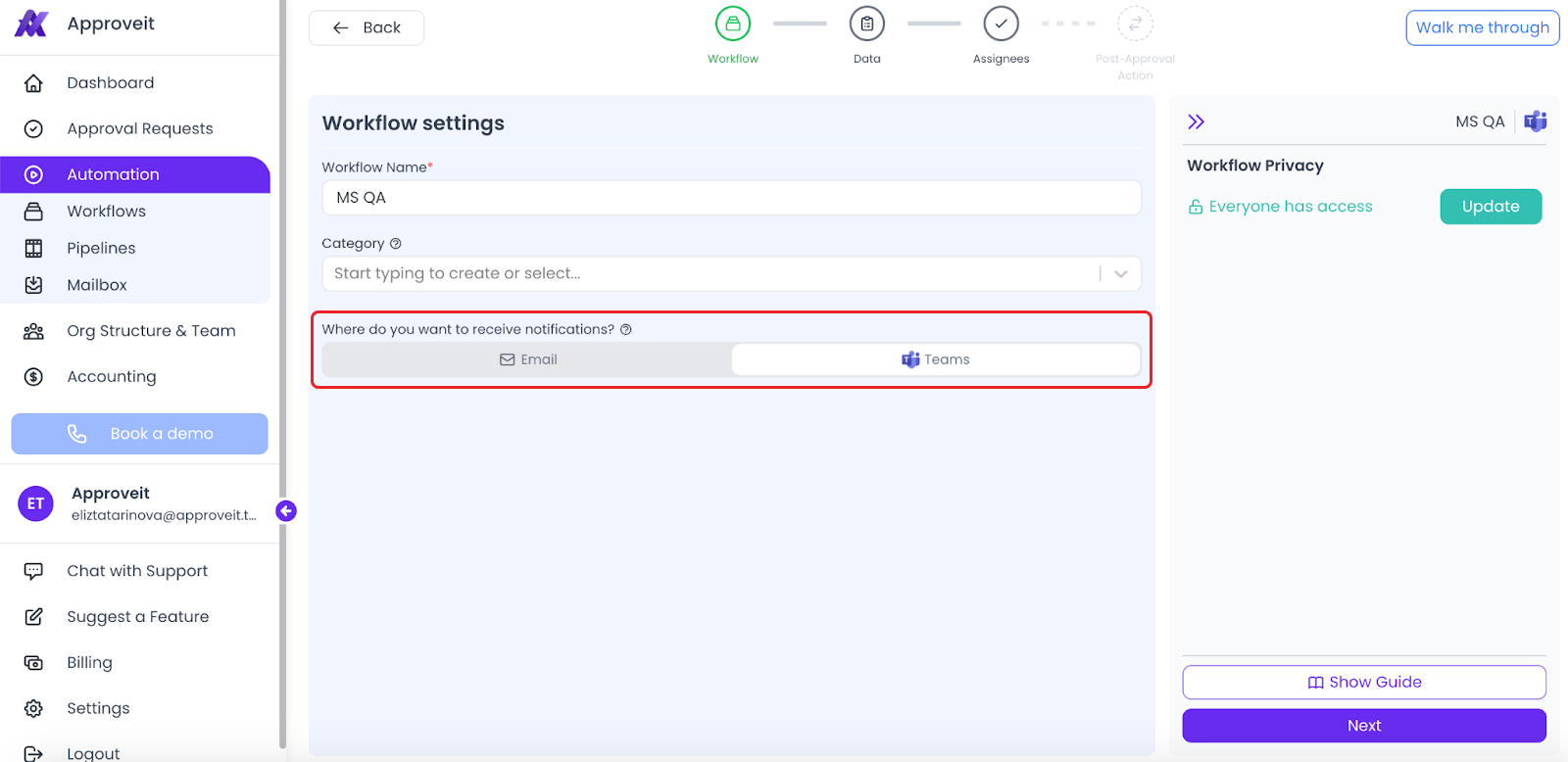This image is a detailed screenshot of an application called "Approve-It." The app features a clean and intuitive interface. The prominent sidebar on the left starts with the app's name, "Approve-It," accompanied by a clever logo where the crossbar of the stylized letter 'A' is a check mark. 

The sidebar menu includes multiple options: 
- Dashboard
- Approval Requests
- Automation
- Workflows
- Pipelines
- Mailbox
- Organizational Structure and Team
- Accounting

Below these options, there are additional links for:
- Chat with Support
- Suggest a Feature
- Billing
- Settings
- Logout

On the main page, the header reads "Workflow Settings." Towards the bottom of this page, there is a red rectangle containing a question about where users want to receive notifications. The text reads "Where do you want to receive notifications?" The available options include "Email" and "Teams," with the "Email" option currently selected.